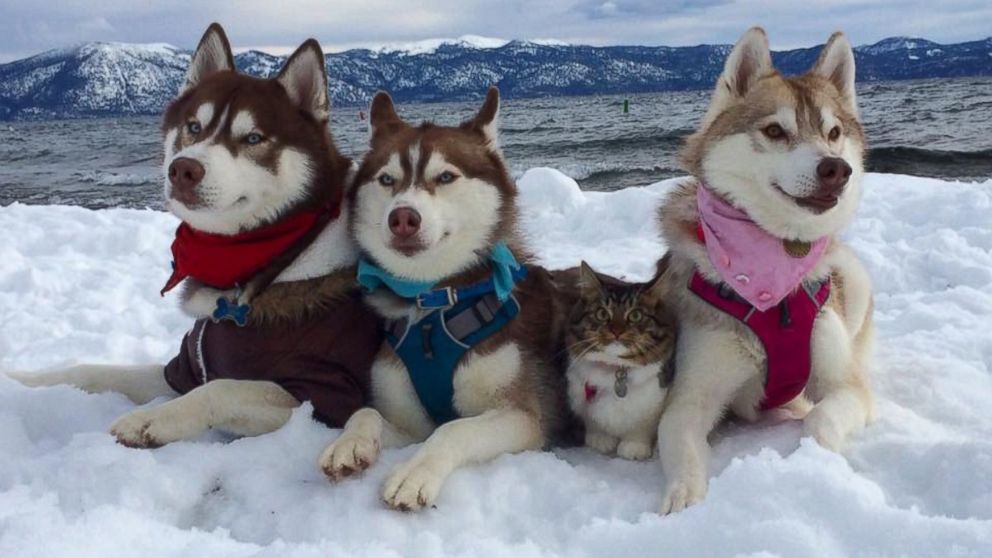In this enchanting image, three husky-type sled dogs and a cat are posing on a floating sheet of ice, possibly in a region like Alaska with visible polar ice caps. The largest of the huskies, positioned on the left, has a striking brown head, piercing light blue eyes, a red bandana, and a blue metal dog tag on its collar. To its right, there is a smaller husky resembling the first but distinguished by a blue collar. Between this smaller husky and another husky on the far right—this one sporting a light tan and white coat with dark eyes—sits an adorable cat with tan, black, and white markings and vivid green eyes. The animals appear to be juveniles, not quite puppies nor fully mature. They are all adorned with harnesses and collars on a snowy icy surface, with majestic snow-capped mountains forming a breathtaking backdrop. The cat, nestled contentedly among the dogs, has an almost inquisitive look, adding a touch of whimsy to this captivating Arctic scene.